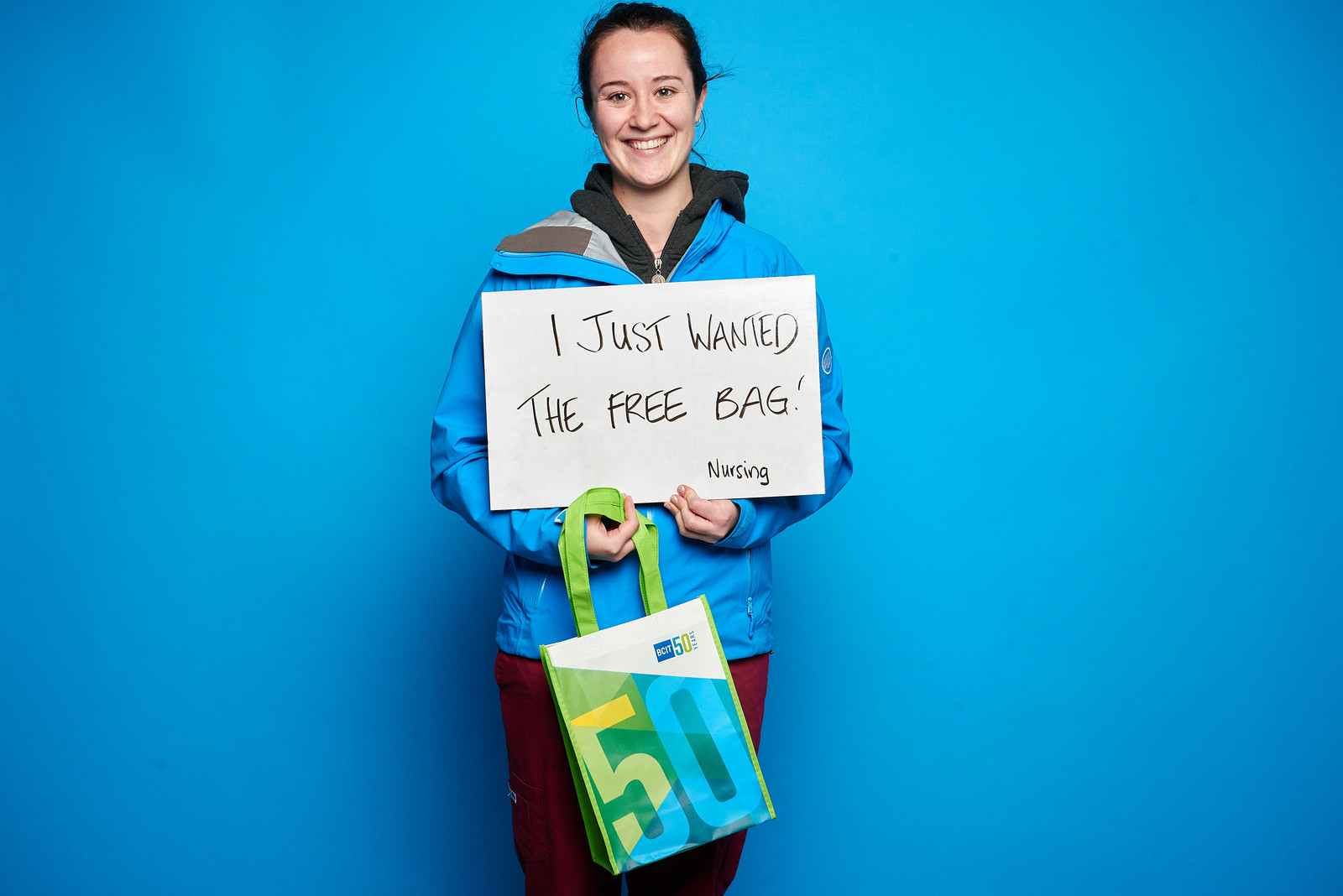In this vibrant photograph, a smiling woman with light skin and dark hair pulled back stands centered against a matte robin's egg blue background. She is wearing a blue zip-up jacket with a white to gray inner lining that extends to her upper thighs, paired with red scrub-style pants. Her dark eyes meet the camera directly, exuding warmth and approachability.

She holds a white rectangular sign across her chest with her hands positioned underneath it. The sign, marked with black letters, reads, "I just wanted the free bag," with the word "Nursing" inscribed in smaller letters below. In her right hand, she clutches a fabric shopping bag featuring a lime green handle. The bag prominently displays the number "50" across its front in large characters. The "5" is primarily white with yellow at the top right and blue at the bottom, while the "0" is in a color matching the photo's background. Lime green and other green shades form the backdrop behind the number. Additionally, though partially obscured, there is text on the bag, seemingly including the characters "CP" followed by "50."